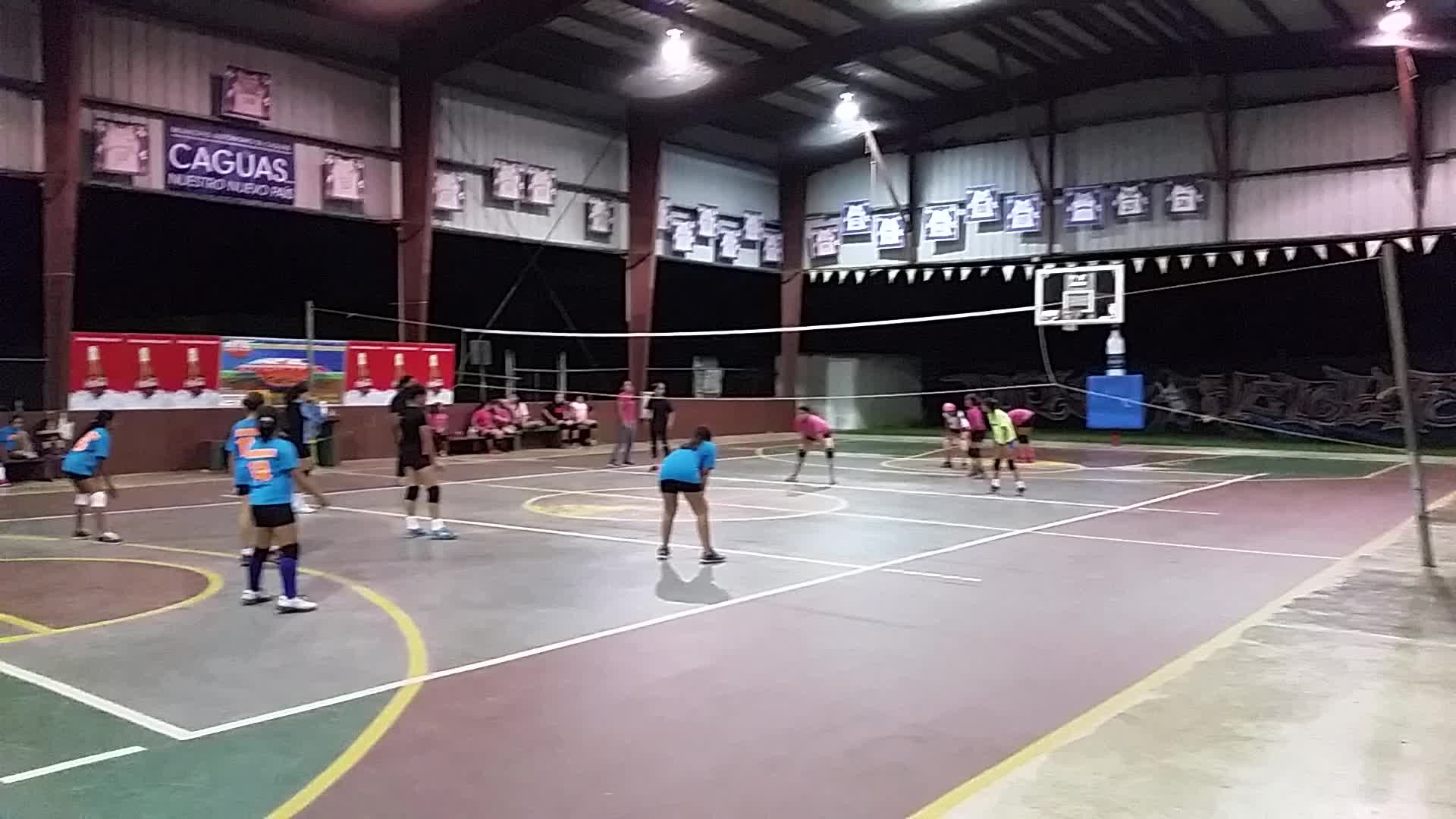This photograph captures a junior high girls' volleyball game in a large, indoor gymnasium with soaring ceilings, akin to an open-structured warehouse, giving it a semi-outdoor feel. The volleyball court, which appears to be laid out on a basketball court, is flanked by two teams: one in light blue shirts and black shorts, and the other in pink shirts and black shorts, with one player in a yellow shirt. The gym’s interior is adorned with banners in Spanish, including "Juegas Nuestro," and equipped with basketball hoops. The players are mostly stationary, with some crouching in preparation while others stand upright, indicating they are gearing up for the next play. Along the court's perimeter, spectators sit on benches, attentively watching the imminent serve from the pink team.